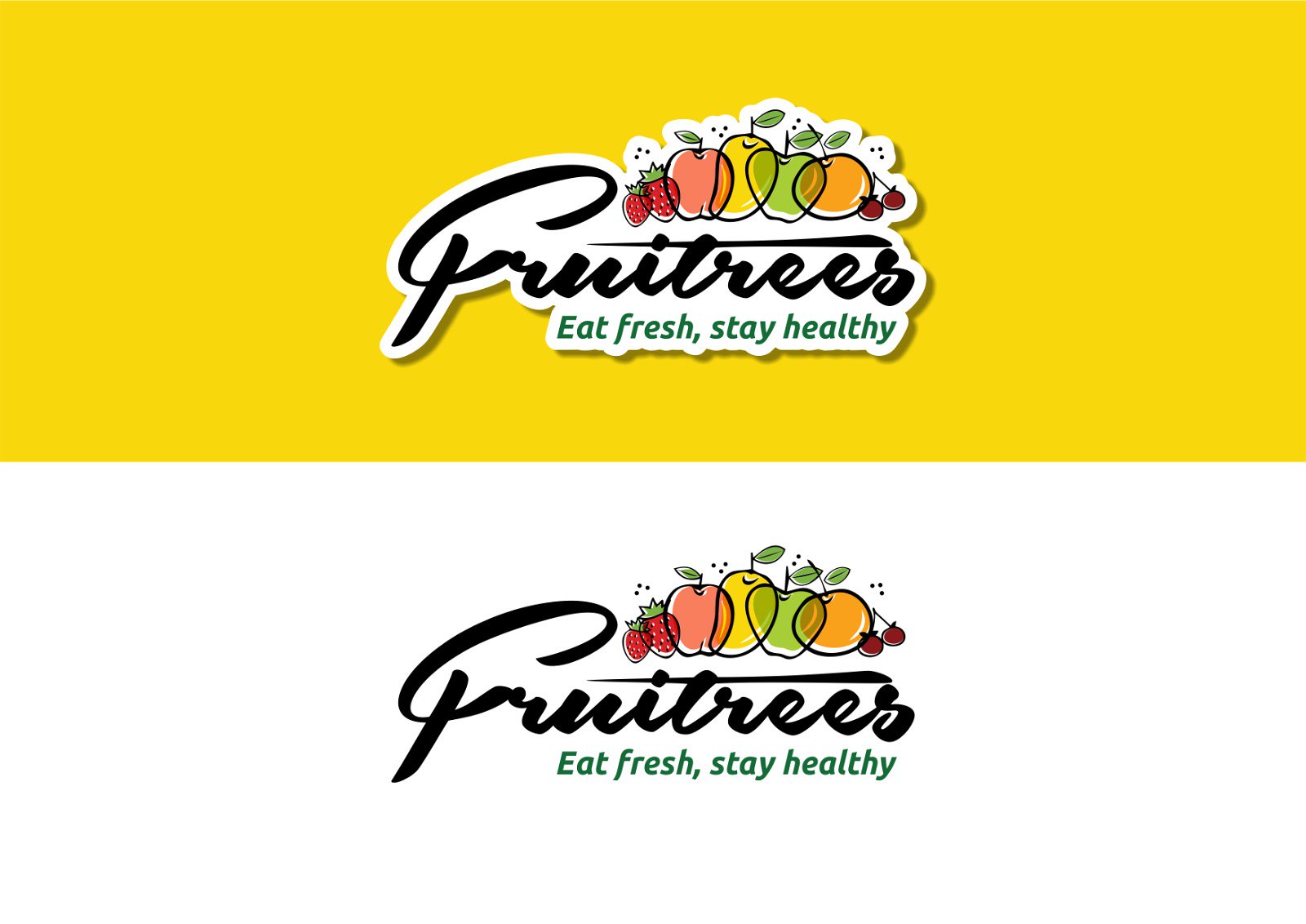The image showcases a vibrant logo for a company named "Fruit Trees." The logo is depicted twice: the top half features the design on a rich yellow background while the bottom half displays it on a plain white background. In both instances, the logo itself consists of the words "Fruit Trees," written in elegant black cursive, with the tagline "Eat Fresh, Stay Healthy" displayed in green underneath. Above the text, there is a whimsical and colorful illustration of various fruits, including strawberries, apples, pears, peaches, oranges, and cherries, all outlined in black. The top version of the image includes an additional pattern that enhances the logo against the yellow backdrop, making it pop, whereas the bottom version presents the logo starkly against the white, emphasizing its clean and fresh design.